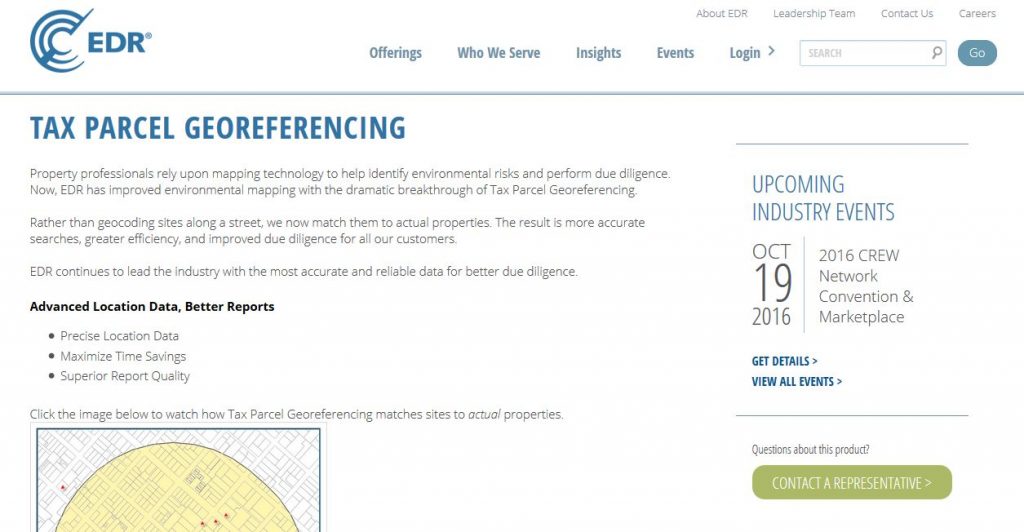The screenshot from EDR highlights a webpage focused on tax parcel geo-referencing. At the top of the webpage are navigation options including Offerings, Who We Serve, Insights, Events, and Login, along with links to Contact Us, Careers, Leadership Team, About EDR, and a search function. The main content details how EDR's advanced mapping technology helps property professionals identify environmental risks and perform due diligence through tax parcel geo-referencing, which provides enhanced location data and superior reports. The page also features a contact option and a highlighted industry event on October 19th, 2016—the Crew Network Convention and Marketplace—with links for further details and a list of all events.